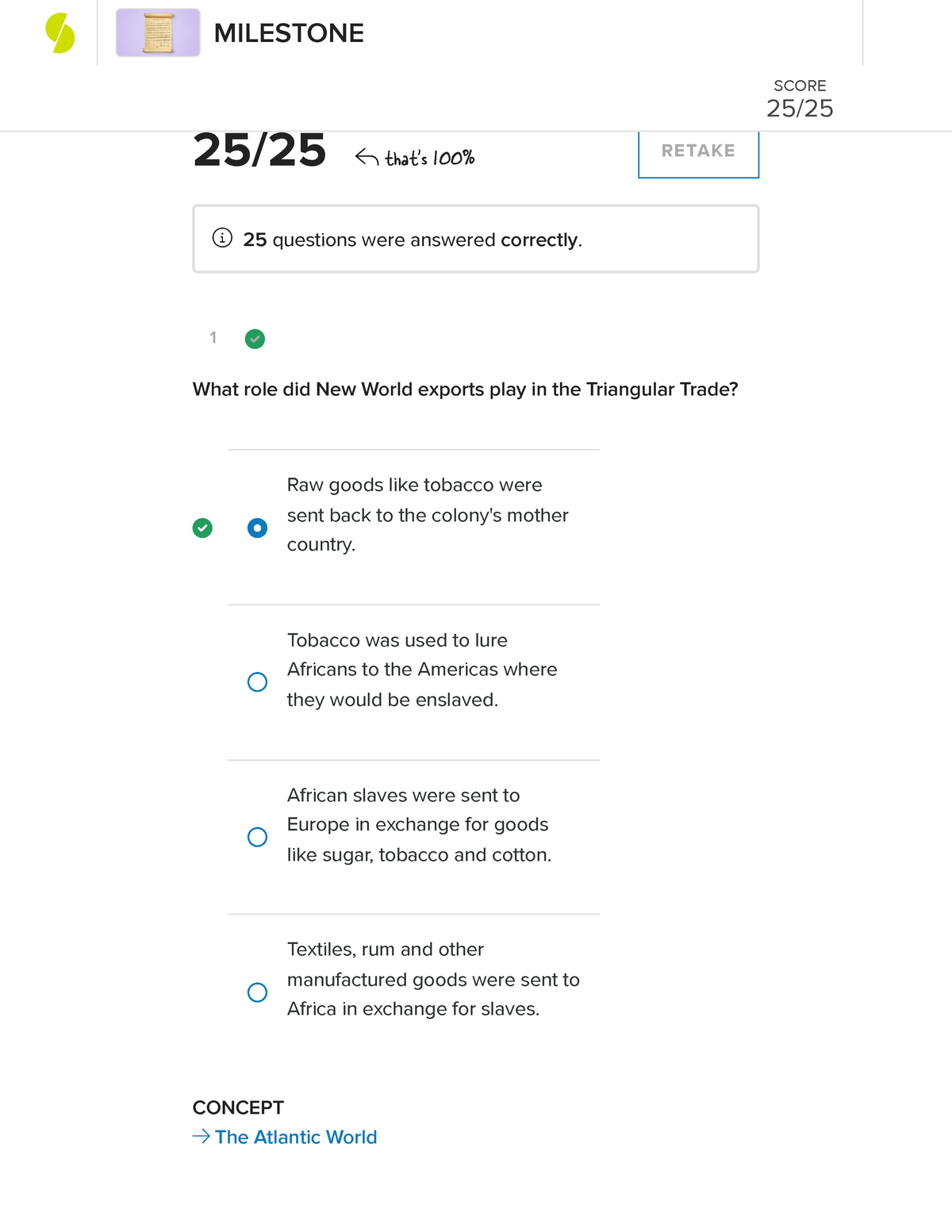The image displays a milestone achievement screen with a detailed breakdown of quiz results. In the top left corner, the word "Milestone" is prominently displayed, followed by an image of a page colored brown with black text set against a purple background. On the top right, an icon depicting a circular shape split in half to form an 'S', with a vibrant green hue, is visible. 

Below the "Milestone" heading, on the top right, the text reads "25 of 25," indicating the total questions answered, and this is reiterated at the bottom of the milestone, emphasizing "25 of 25, that's 100%". Additionally, a "Retake" button is situated on the right side.

At the bottom, the text states that "25 questions were answered correctly." Following that, there is a question: "What role did New World exports play in the triangular trade?" with multiple bullet points listing possible answers:

1. Raw goods like tobacco were sent back to the colonies.
2. Tobacco was used to lure Africans to the Americas where they would be enslaved.
3. African slaves were sent to Europe in exchange for goods like sugar, tobacco, and cotton.
4. Textiles, rum, and other manufactured goods were sent to Africa in exchange for slaves.

The first answer, "Raw goods like tobacco were sent back to the colonies," is highlighted in blue and marked with a green tick to denote it as the correct response.

On the bottom left, the term "Concept" is shown with "The Atlantic World" written in blue beside it, against the word "Concept" in black.